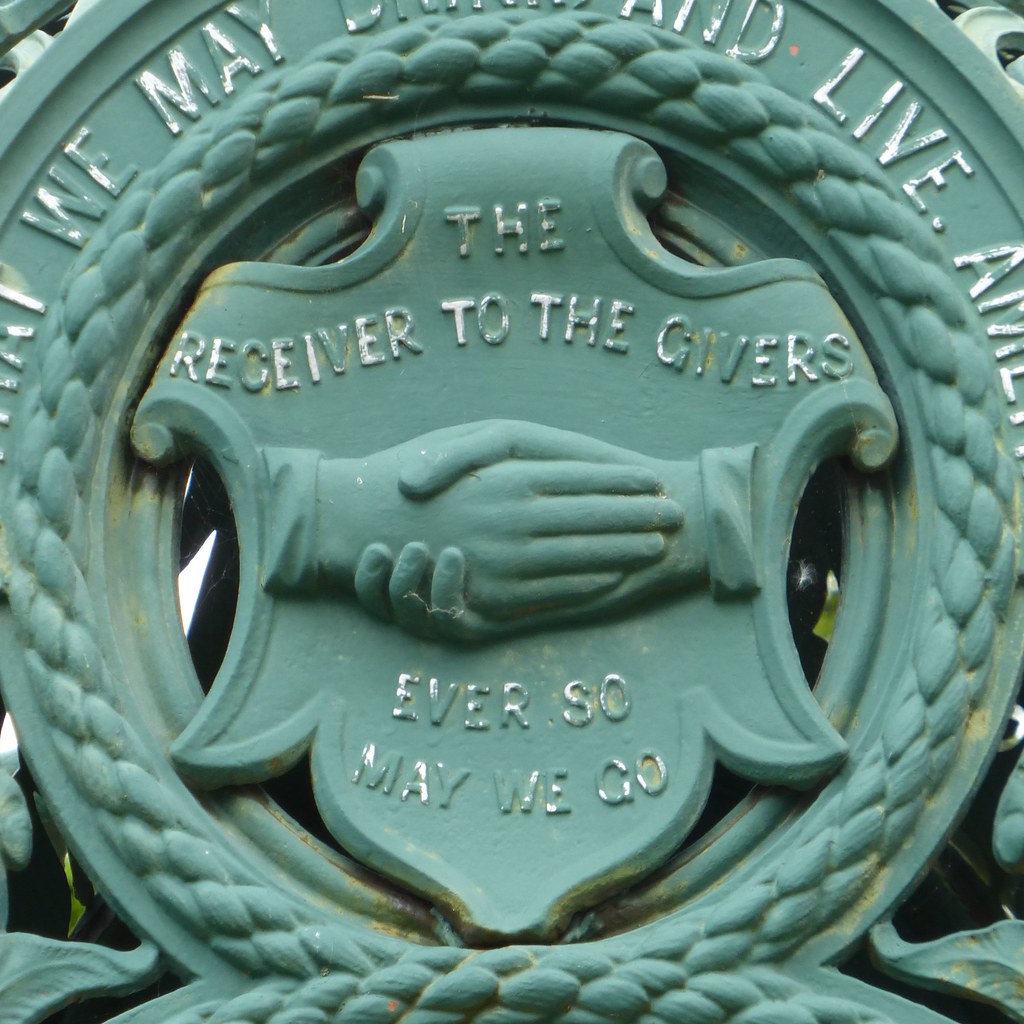This image features a weathered green cast plaque, likely made of metal or stone, adorned with intricate details and inscriptions. In the center of the plaque, there is a motif of two hands clasped in a handshake, symbolizing unity or agreement. Surrounding the handshake is a circular braided wreath, meticulously textured to resemble rope. Above and below the central handshake, there are distinct inscriptions: "The receiver to the givers" at the top and "Ever so may we go" at the bottom. An additional circular border of text encircles the wreath, although parts of it are faded and difficult to decipher; the legible portions include the words "we may" and "live." The entire plaque, in a pale green color that has faded to yellow in some areas due to its age, shows signs of wear with rough spots and peeling white lettering. The background of the image is faintly white, providing no significant distractions from the plaque itself. The plaque appears outdoors, secured to what might be a chair or bench, as suggested by the presence of metallic elements.